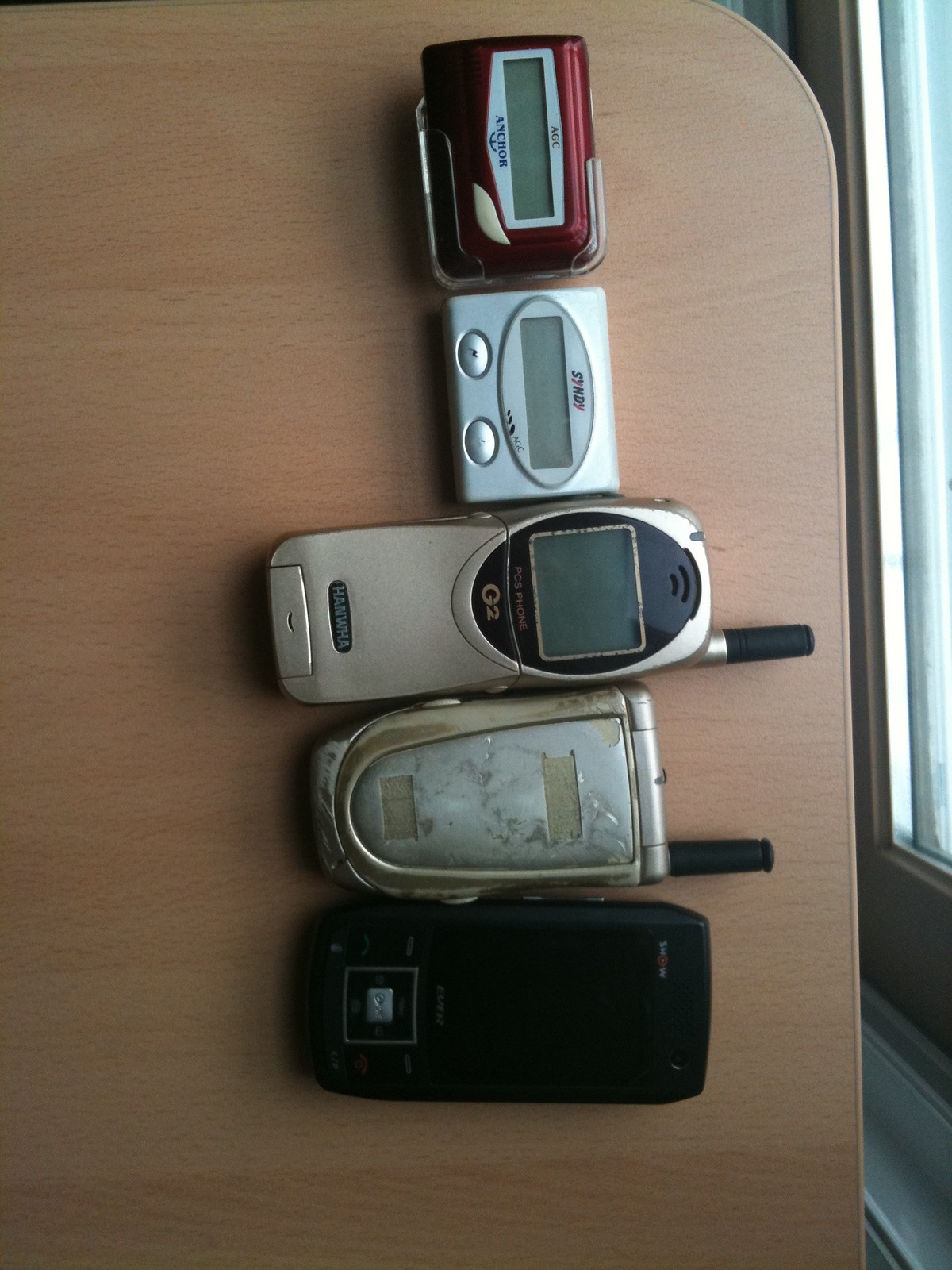A detailed aerial photograph captures a line of vintage communication devices arranged vertically on a light brown wooden surface. The sequence begins at the top with a red rectangular pager featuring a white button and the brand name "Anchor" below its screen. Just below it lies a silver pager marked with the brand "SYNDY," characterized by its compact size and two oval buttons. Beneath the pagers, the next device is an elongated silver cell phone with a black antenna and a screen displaying "PCS Phone G2 Hanwha." Following this is a heavily worn silver flip phone with visible scuffs and a bulky antenna. At the very bottom is a sleek, modern-era black flip phone, devoid of an antenna and featuring a subtle silver button. To the right, a window allows a soft blue-white light to spill onto the devices, casting gentle shadows and adding depth to the image.